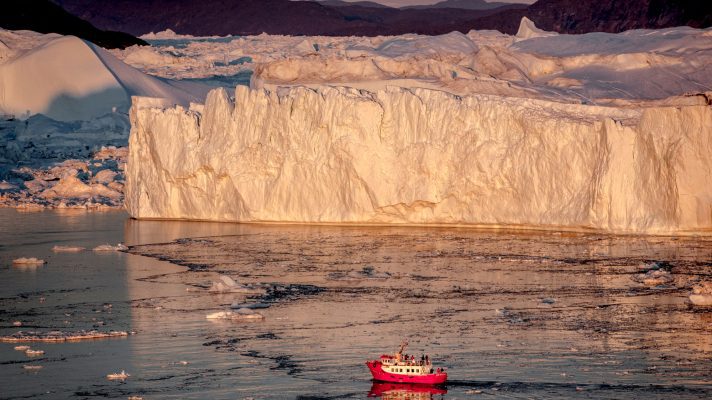The photograph captures a breathtaking outdoor scene likely set in Alaska or the Arctic. Dominating the top portion of the image is a monumental, pyramid-shaped iceberg, radiant in the sunlight, with its towering, white, straight-sided presence gleaming against the sky. The scene appears to be bathed in the warm hues of a sunset, casting an enchanting orange glow on the snow and ice-covered land. 

Floating in the extensive body of clear, icy water are clusters of smaller ice chunks. Nestled in this aquatic expanse is a red and white boat, which, despite having approximately ten people on its deck, looks astonishingly tiny against the colossal iceberg. The boat’s passengers are minuscule, barely noticeable at this scale. The boat is heading to the left and is the only vessel present in this pristine, glacial seascape, accentuating the vast, untouched beauty of this frozen wilderness. The overall clarity of the image is exceptional, capturing the bright, natural light of the daytime, which accentuates the vivid details of the landscape.